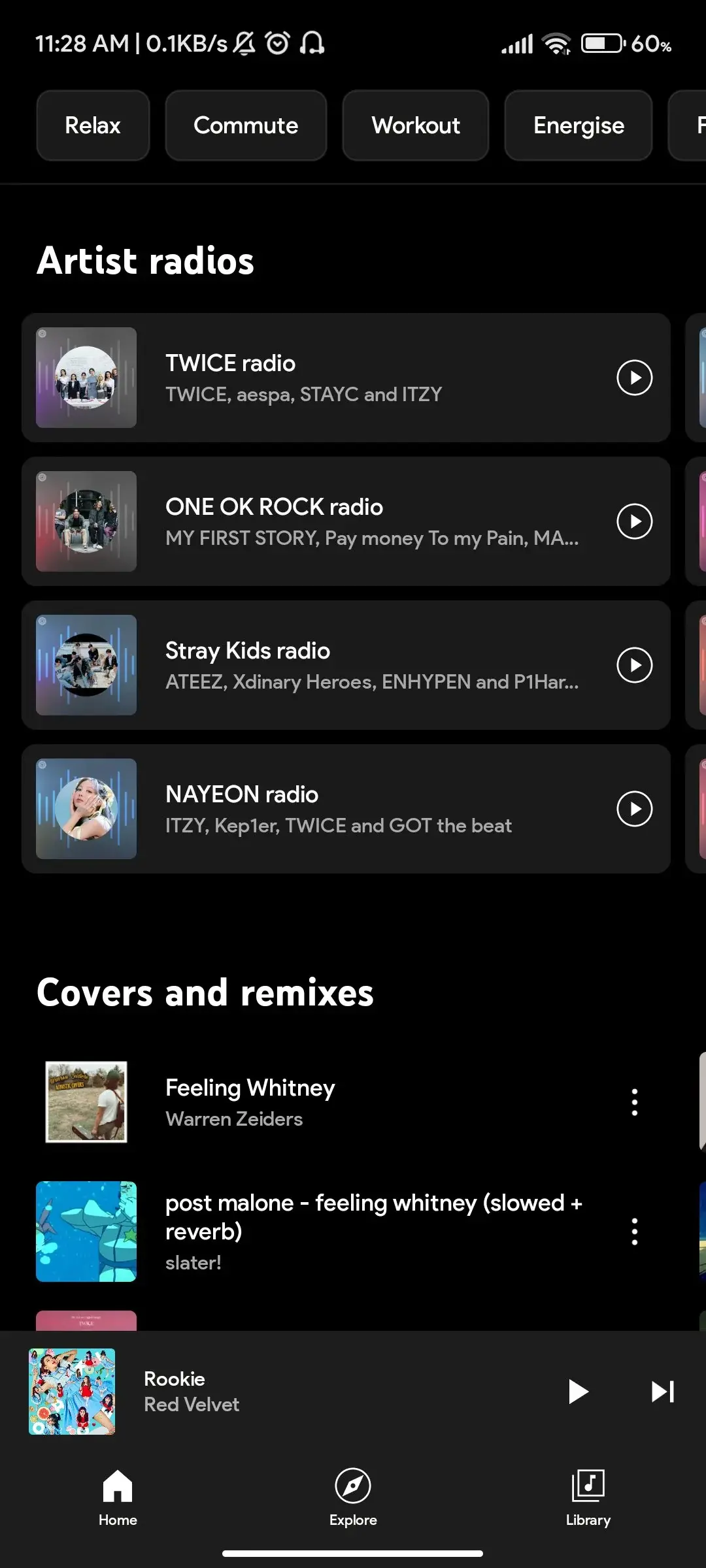A detailed screenshot of a smartphone display shows a user browsing a radio streaming website. The screen timestamp at the top reads 11:28 AM, with bell notifications turned off and full Wi-Fi signal strength indicated. The device's volume is set to approximately 75%, and the battery is at 60%. 

The content in view includes a section titled "Artist Radios," offering four radio station options for different artists. Below this, a category labeled "Covers and Remixes" lists specific tracks like "Feeling Whitney" by Warren Zeiders and an option for Post Malone. A prominent gray button below these options provides another selection labeled "Rookie."

Navigation controls are present at the screen's bottom, featuring buttons for Home, Explore, and Library. The selection areas for the stations stand out in dark gray, set against the black background of the site, emphasizing a sleek and modern interface.